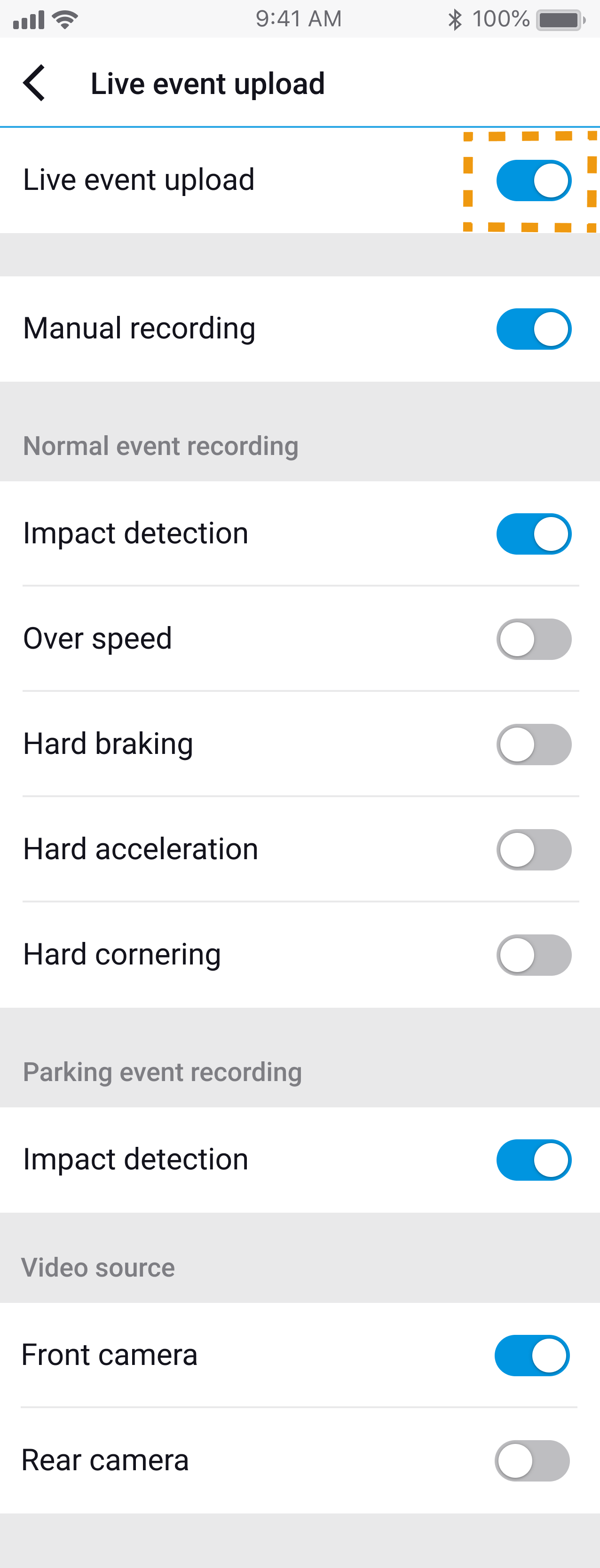Screenshot of a Mobile App Interface Displaying Various Event Upload Options with Toggle Buttons.

The screenshot captures the interface of a mobile application titled "Live Event Upload." The screen is divided into four distinct sections, each separated by gray lines. At the top of the screen, the title "Live Event Upload" is prominently displayed in bold text, accompanied by a dashed orange square surrounding it to highlight its importance. Below the title, there are several toggle buttons that control different features of the app. These buttons indicate their status through color coding: blue for active (on) and gray for inactive (off).

The options are organized into three groups under the main title. The detailed breakdown is as follows:

1. **Group 1:**
   - **Manual Recordings:** Toggled on, indicated by a blue switch.
   - **Impact Detection:** Toggled on, indicated by a blue switch.

2. **Group 2:**
   - **Over Speed:** Toggled off, indicated by a gray switch.
   - **Hard Braking:** Toggled off, indicated by a gray switch.
   - **Hard Acceleration:** Toggled off, indicated by a gray switch.
   - **Hard Cornering:** Toggled off, indicated by a gray switch.

3. **Group 3:**
   - **Impact Detection:** Toggled on, indicated by a blue switch.
   - **Front Camera:** Toggled on, indicated by a blue switch.
   - **Rear Camera:** Toggled off, indicated by a gray switch.

At the top of the screen, the phone's user interface is visible, showing the remaining battery life and other standard icons.

This detailed view provides a comprehensive overview of the app's event upload settings, allowing users to easily manage their preferences for recording and detecting various events.